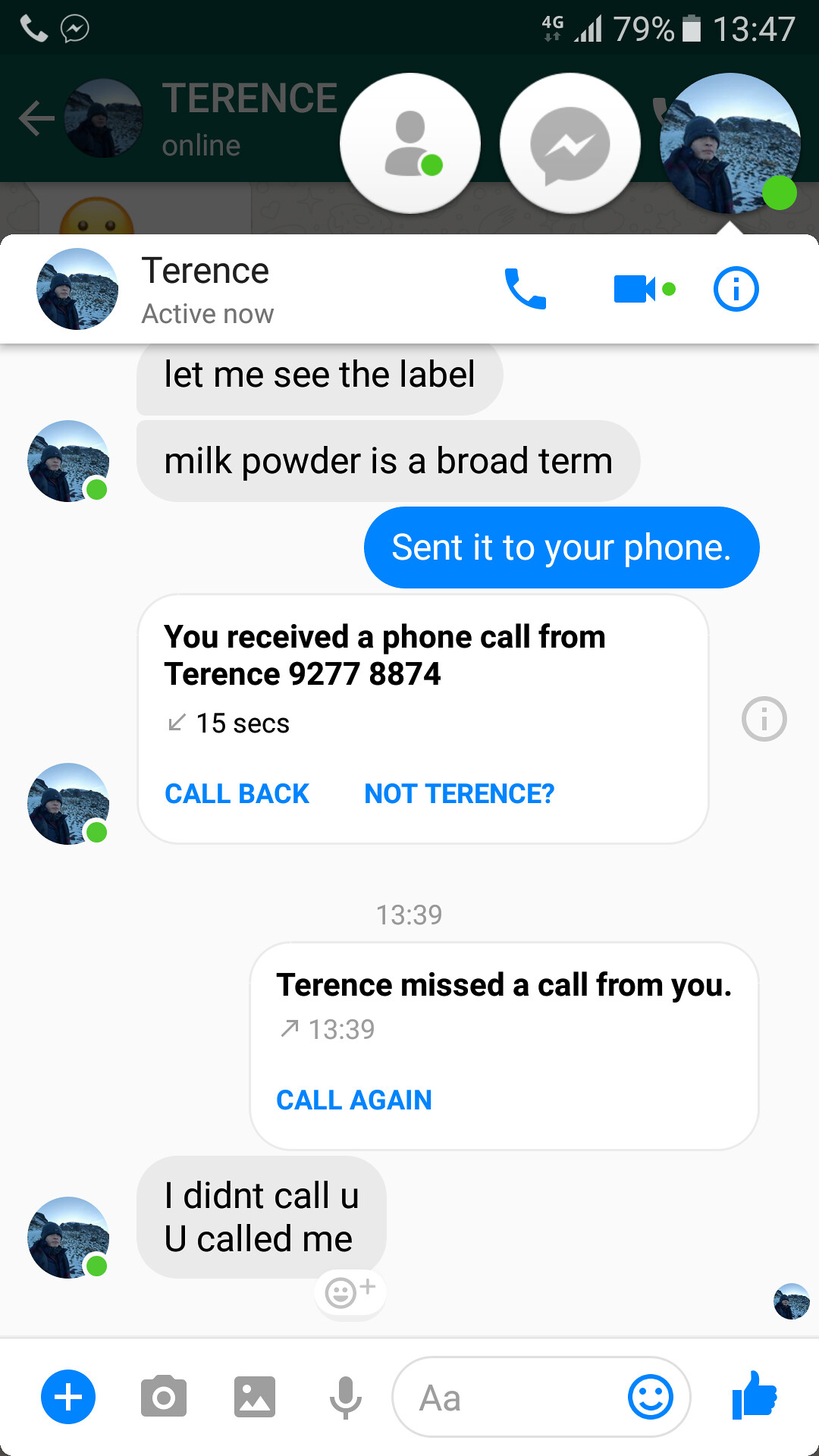This image is a detailed screenshot of a cellphone displaying a messaging app conversation with a person named Terence. The phone, showing a 79% battery level, 4G connection, three or four signal bars, and the time stamp of 13:47, has multiple icons visible at the top: a phone symbol on the upper left, and indicators for battery, power, and Wi-Fi on the upper right. Terence's name is prominently displayed at the top of the screen, appearing faintly in gray on a black background, accompanied by status "active now" and his avatar—a profile image depicting Terence against a hill with a blue sky.

The messaging app interface features various icons including a telephone, a video camera, and an information symbol. The conversation displayed begins with Terence messaging, "Let me see the label. Milk powder is a broad term." The user replies, "Sent it to your phone." Following this, a notification within the conversation states, "You received a phone call from Terence," accompanied by the phone number 9277 8874. Beneath this is the option to "Call back" or select "Not Terence". At 13:39, another message indicates, "Terence missed a call from you. Call again." Terence responds, "I didn't call you, you called me," written informally as, "I didn't call u, u called me," alongside a smiley face emoji with a plus sign.

Situated at the bottom of the screen are icons for a plus sign, a camera, a landscape image, a microphone, a text input box labeled with "Aa", and a smiley face emoji. Additionally, there is a separate thumbs-up icon in blue. This comprehensive screenshot meticulously captures the details of the ongoing chat between the user and Terence, alongside the phone's status information.